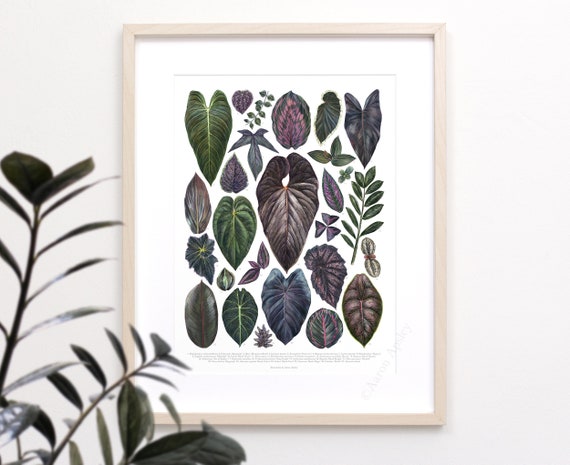The image features a framed botanical portrait hanging on a wall painted in a very light gray, almost white shade, which contrasts subtly with the brighter white of the print. The portrait showcases a variety of illustrated leaves, meticulously organized in rows. The leaves exhibit a spectrum of colors, including various shades of green, blue, purple, and violet, and come in diverse shapes and sizes—some large, others small and skinny, some attached to stems. Notable leaves include a heart-shaped purple leaf in the upper right, a black leaf in the upper left, a palm-shaped green leaf, a turtle shell-like leaf in the bottom right, and a waxy-looking leaf in the bottom left. The artwork is set within a light wood frame, almost whitewashed, with a white matte border that elegantly frames the white background of the print. In the foreground, to the lower left of the portrait, there stands a tall plant with green leaves, creating a visual echo of the botanical theme in the portrait.